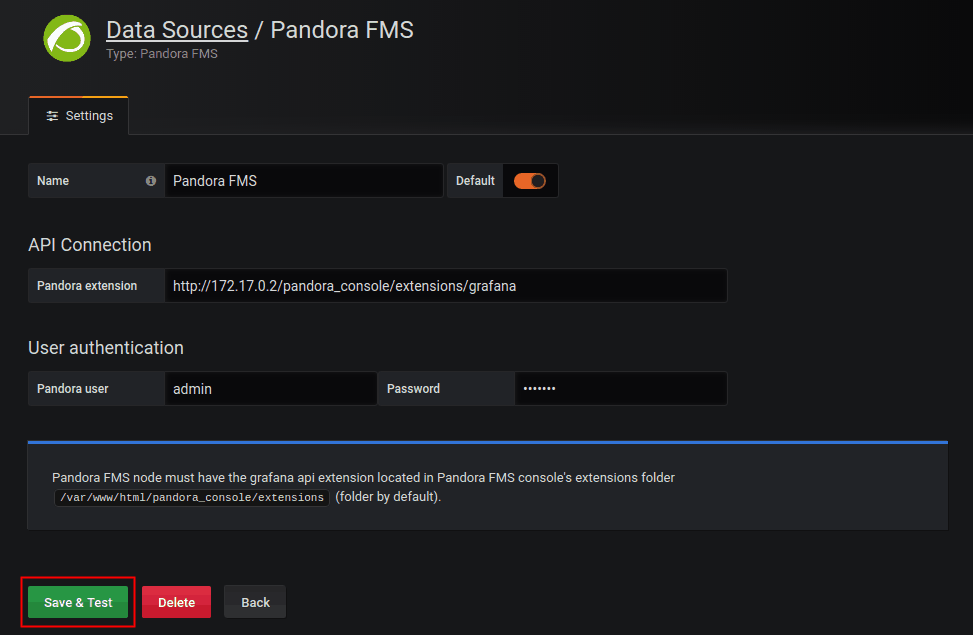The image features a black background with a green circle positioned at the top left corner. Inside the green circle, there is a logo that comprises a central circle and a banner across the top, though its exact design is not specified. The logo is accompanied by the text "Data Sources / Pandora FMS" with "Pandora FMS" highlighted.

Beneath this, an orange line displays the sentence "Name: Pandora FMS Default," followed by an orange button labeled "Turn On Default Setting."

Further down, there is a section titled "API Connection" with the following URL: "http://172.17.0.2/pandora_console/extension/grafana."

Below this, the user authentication details are mentioned: "Pandora User: admin," with the password field obscured. 

Finally, a note indicates, "Pandora FMS mode must have the Grafana API extension located in the Pandora FMS console extension folder."